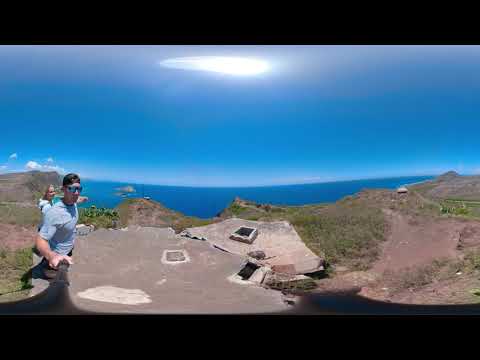This outdoor photograph captures a stunning natural landscape from what appears to be the top of a hill or a mountain. The image foreground displays two people, both on the left side: a man and a woman. The man, wearing a light blue t-shirt, dark rimmed sunglasses with bright blue lenses, and a backward hat, is holding a selfie stick to capture the panoramic view. He is facing the camera, showing a three-quarter profile, with his right arm bent, probably resting in his pocket. Behind him stands a blonde woman, partially obscured by the man, dressed in a light blue or white jacket. The photograph showcases the brilliant blue ocean in the background, meeting a flat horizon marked by a vibrant blue sky. The sky features the sun centered just above the horizon, casting beautiful light across the scene. The ground around them consists of dirt, rocky surfaces, and patches of grass, with the entire setting bathed in natural sunlight. The view is expansive, featuring rolling hills or a grassy expanse lying between their elevated position and the distant horizon, creating a breathtaking, almost serene landscape.